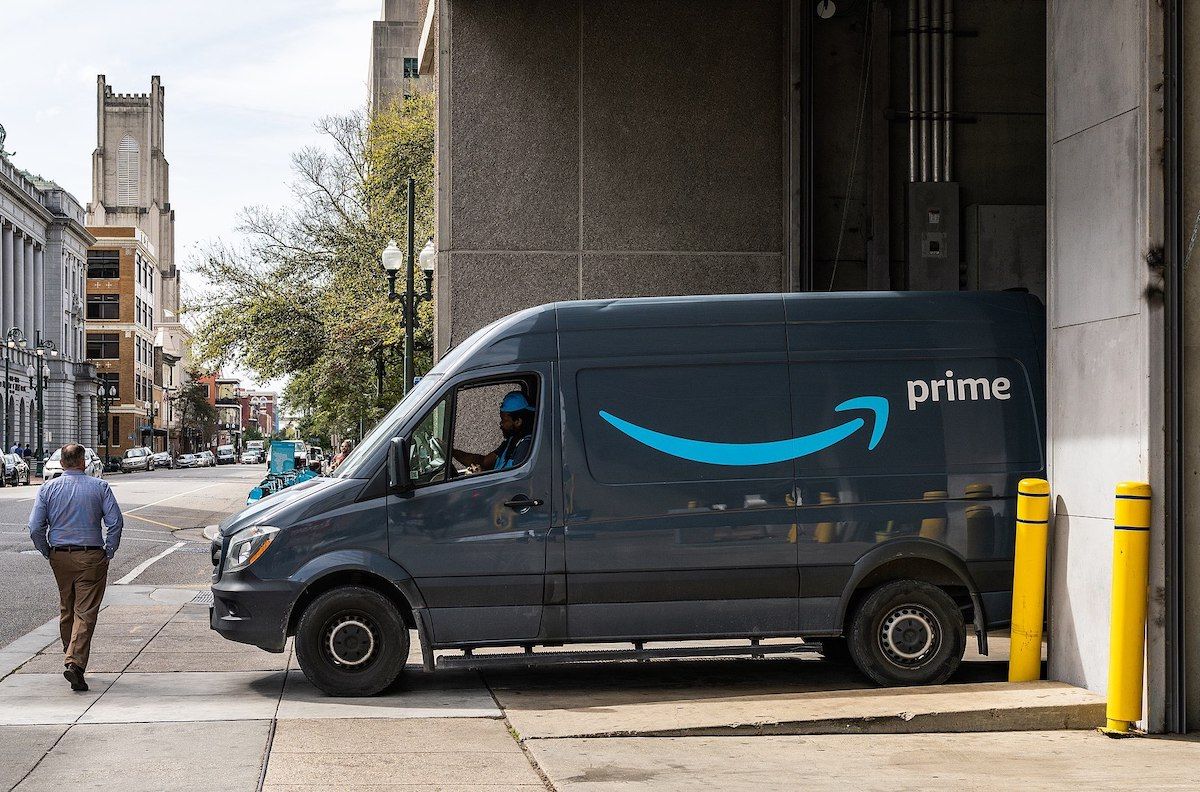The outdoor scene captures a bustling urban street against a predominantly blue sky, lightly veiled with scattered clouds. Dominating the left side of the image, various buildings of gray, brown, red, and tan hues rise to relatively uniform heights, with the exception of a central structure distinguished by a towering spire. Below these buildings, a row of cars lines the street, juxtaposed by several more buildings on the opposite side, with one prominent gray building anchoring the mid-ground.

At the forefront of this urban tableau, a sidewalk hosts a lamppost and a pedestrian—a man clad in a blue long-sleeve shirt, brown pants, and dark brown shoes, walking with his hands in his pockets. A striking blue Amazon van, featuring a light blue, upward-pointing arrow and the word "Prime" inscribed in white letters, is parked nearby. The van's driver, sporting a backwards baseball cap, is visible through the side window. Adding to the metropolitan details, two yellow poles stand beside the building adjacent to the van, completing the vibrant city scene.